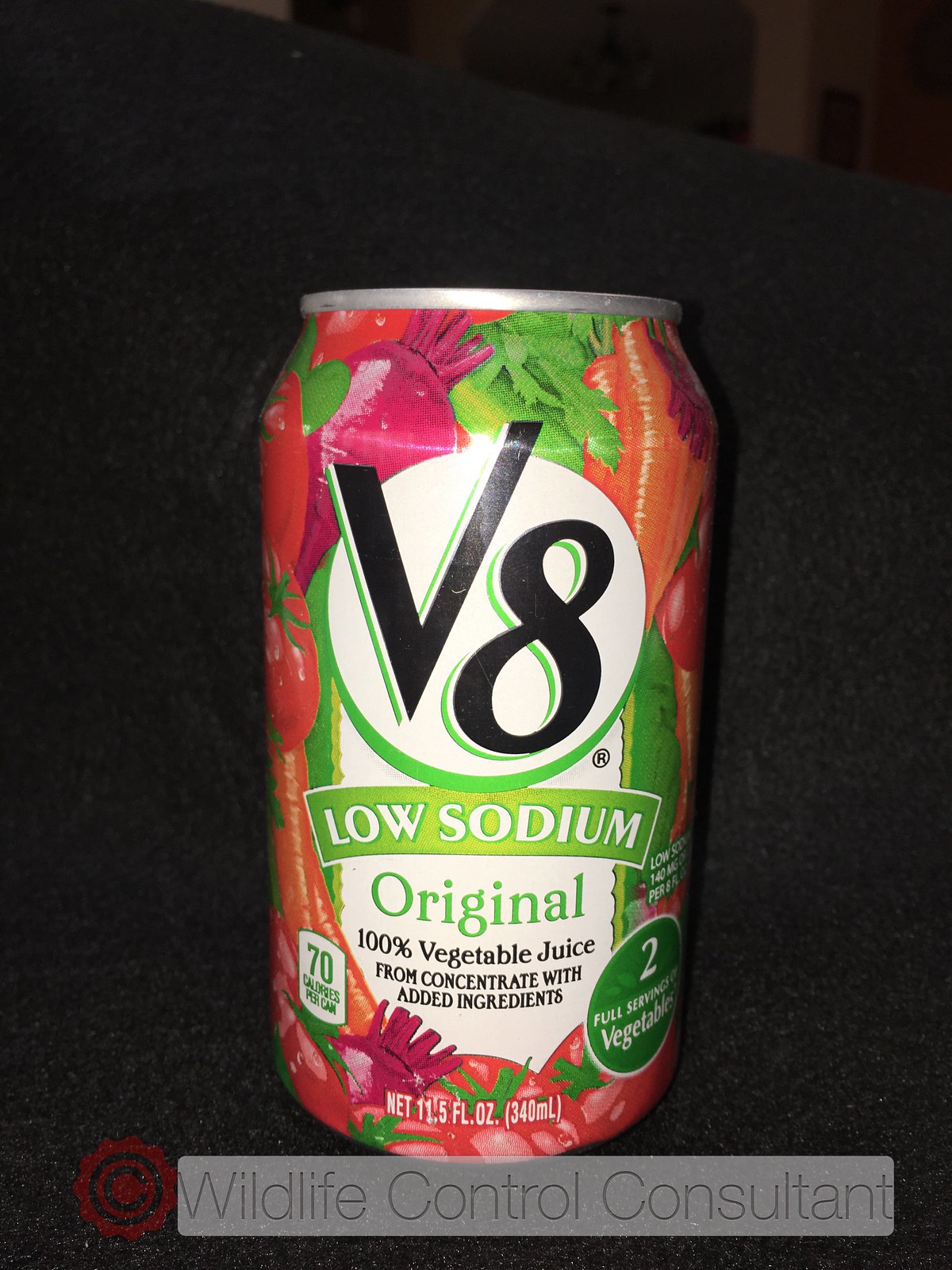This image is a detailed photograph of a can of V8 juice, prominently showcasing its features. The aluminum can is labeled "V8 Low Sodium Original 100% Vegetable Juice from Concentrate with Added Ingredients." It contains 11.5 fluid ounces (340 milliliters) of juice and provides 70 calories per can. The design on the can includes vibrant images of vegetables such as orange carrots, red tomatoes, purple beets, and green celery with other leafy greens. The front of the can features the V8 logo in black lettering with a green outline, set within a white circle that also has a green outline. The words "low sodium" are written in white on a green banner, while "original" is displayed in green on a white background. A green circle on the right-hand side claims "two full servings of vegetables," and there's a standard calorie logo on the left side indicating the caloric content. At the bottom of the can, there is an unexpected watermark with a copyright symbol stating "wildlife control consultant," though no other details in the image connect it to wildlife control. The can is positioned on a dark piece of foam or a similar surface, and the background is also dark, highlighting the can's vibrant design. The top of the can is not visible, so it is unclear if it is open or closed.